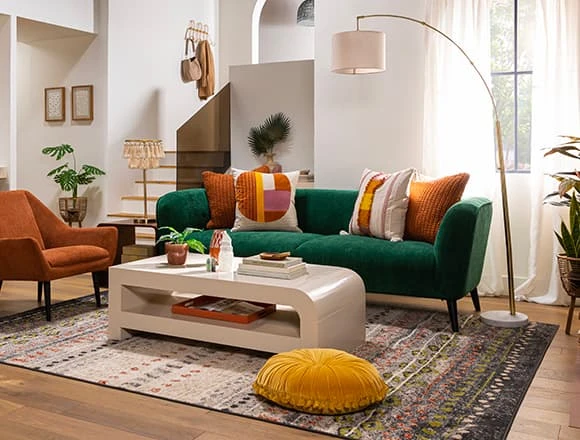The living room, bathed in natural daylight, features a harmonious blend of colors and textures. Dominating the scene is a plush green couch adorned with an assortment of pillows in brown, lavender with designs, and beige. Adjacent to the couch on the left is a inviting brown chair, both set on a hardwood floor. The central area showcases a white, rounded coffee table, its surface and lower shelf layered with various items, all resting on a patterned rug in hues of gray, purple, and white.

A notable detail is the round, mustard-colored cushion placed casually on the floor, adding a touch of whimsy. To the right of the couch, a sleek, white floor lamp arcs over with a delicate lampshade, illuminating the cozy corner near a half-open window draped with white curtains.

In the background, the living space extends with a visible staircase ascending to the left of the couch, accompanied by a wall decorated with a couple of framed pictures and a green fern in a vase underneath. Beyond this, there's an opening leading to another room, denoted by a rack holding a brown bag and a coat. Scattered potted plants add a touch of vibrancy, completing the inviting ambiance of this thoughtfully curated living room.